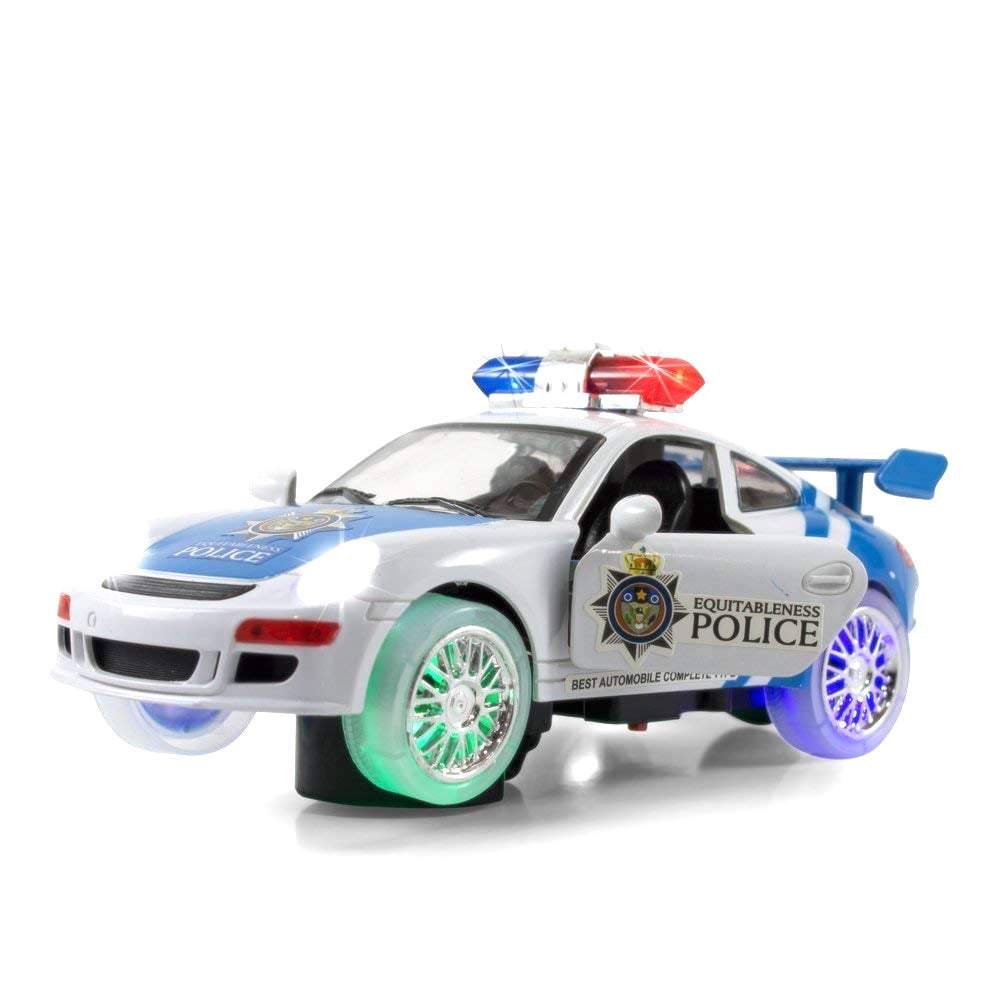This image captures a highly detailed close-up of a plastic toy police car resembling a Porsche. The toy car, primarily white with blue accents, boasts distinct features: a red and blue light bar on the roof, a cyan blue spoiler at the back, and illuminated wheels—green neon light on the front left tire, blue on the back left, and neon-lit green and purple wheels on the right side. The door of the car is open, displaying the text "Equitableness Police" along with a blue, yellow, black, and white logo. The headlights and light bar are also lit, underscoring the car's realism. Mounted on a black stand and tilted slightly to the left, the car features a detailed interior with black seats, windshields on both ends, and side windows. The car's hood is cyan with white patches, and it has blue striping on the back, with the left and right sides differentiated by blue and red colors, respectively, separated by a silver trim. This meticulously crafted toy embodies the quintessential police cruiser aesthetic.